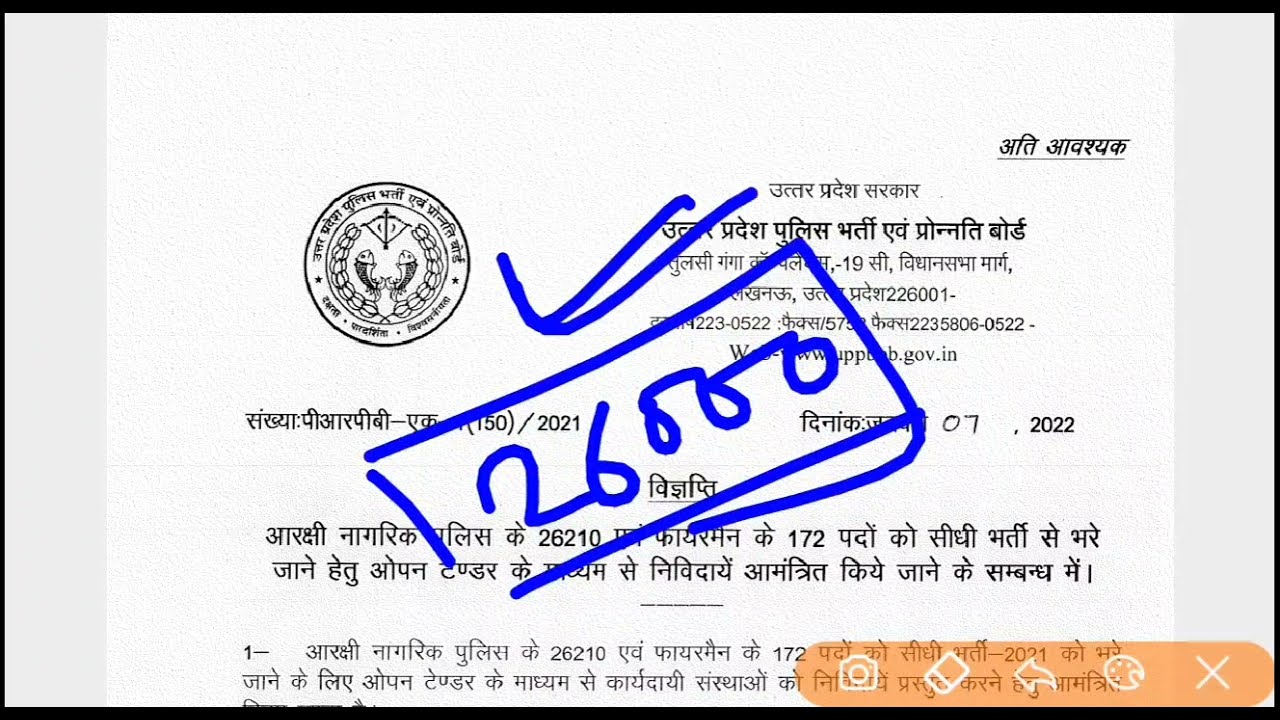The image depicts a white paper document, possibly of a legal or business nature, written in an Indian language. The document features text in black ink, and prominently on the top right is a black circular seal with intricate designs, including text wrapped around its edges and the depiction of two curved fish in the center. Overlaying the document is a blue marker box with the number "26,000" inside it and two blue check marks positioned directly above. In the upper left section, there's a date noted as "07, 2022." The lower portion of the document shows an interface containing icons such as an X, a paint palette, an arrow, an eraser, and a camera, suggesting it might be displayed or edited using image editing software.